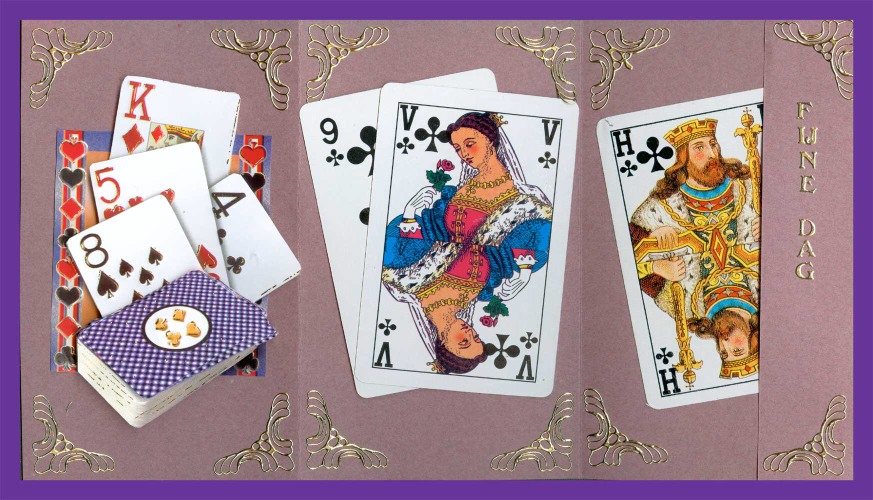The image showcases an intricate paper design with a bold, bright purple border framing a light burgundy background. The burgundy layer appears to be slightly lifted at the bottom left and right corners, suggesting it has been glued over the top. Elegantly adorning each corner are raised designs crafted from gold paint, with four on the top and four on the bottom, evenly spaced for a balanced aesthetic.

On the left side of the design, a stack of playing cards is glued onto the paper, with four cards prominently placed above it. These cards are as follows: the Ace of Spades, the Five of Hearts, the King of Diamonds, and the Four of Clubs, each leaning towards the right. Adjacent to this stack are two more cards, one atop the other: the Nine of Clubs and the Queen of Clubs, recognizable by the queen's illustration on it. The final card on the right is partially obscured by a piece of paper taped over its top, which reads "Thundag." Despite this obstruction, one can discern that the hidden card is either the King of Clubs (as suggested by the letter "H") or another significant face card.